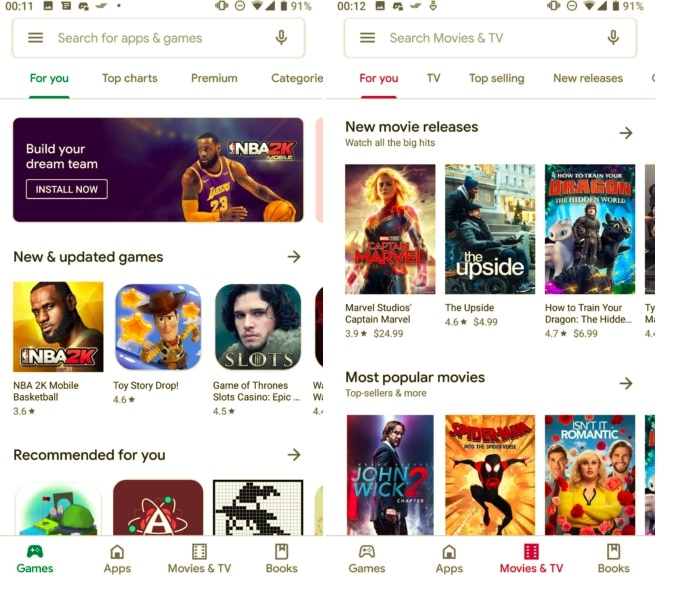The image consists of two sections showcasing cell phone screens. The left section displays a variety of app and game recommendations with the following details:

- **Time and Battery Indicator:** Shows "00:11" and "91%" battery life.
- **Search Header:** Text reads "Search for apps and games for you."
- **Recommendation Highlights:**
  - **Build your dream team. Install now. NBA 2K**
  - **News and updates: NBA 2K**
  - **Toy Story Drop**
  - **Game of Thrones Slots**

At the bottom of this section, there are category tabs labeled "Games," "Apps," "Movies," "TV," and "Books."

The right section focuses on recommended movies and TV shows, featuring:

- **Search Header:** Text reads "Movies and TV for you."
- **New Movies Released:** Includes titles like "Marvel Studio: Captain Marvel," "The Upside," and "How to Train Your Dragon."
- **Most Popular Movies:** Lists "John Wick 2," "Spider-Man," and "Isn't it Romantic?"

Similar to the left section, the bottom displays tabs for "Games," "Apps," "Movies," "TV," and "Books."

The overall color scheme is dynamic and vibrant, featuring a mix of gray, white, green, red, purple, blue, yellow, orange, brown, peach, black, and various other shades, enhancing the visual appeal of the interface.